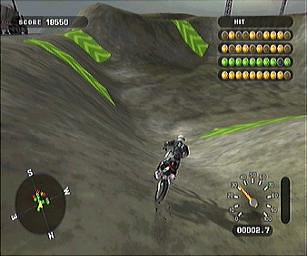The image depicts a dynamic scene from a video game, where a motorcyclist is navigating through a series of undulating dirt hills within a valley. The terrain is rugged, characterized by earthy brown and tan hues that present an off-road challenge. Prominently, there are fluorescent green directional arrows strategically placed on some of the hills, guiding the player on the intended path. These directional markers stand out with their vivid green labels and white arrows, providing clear navigation cues.

In addition to the immersive landscape, the game's interface features several functional overlays. In the upper right-hand corner, there is a scoreboard displaying the player's accumulated points or achievements. The bottom right-hand corner houses a clock, likely used to track time elapsed or time remaining for the mission. To aid in orientation, a compass is situated in the bottom left corner, offering directional guidance. Meanwhile, the score, prominently displayed in the upper left-hand corner, provides real-time feedback on the player's progress and performance.